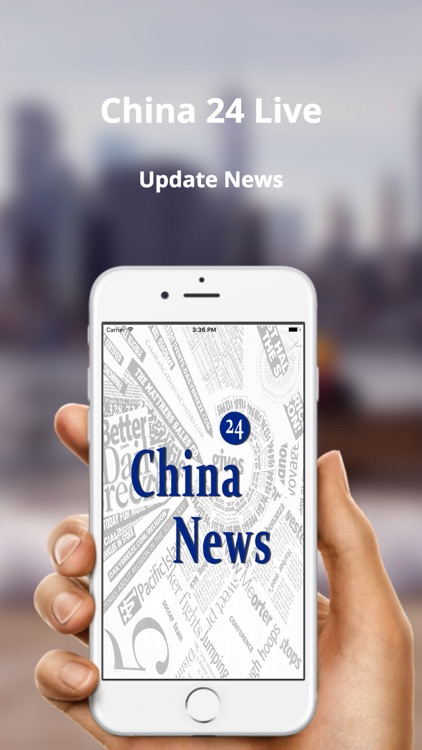The image depicts a hand holding a white iPhone prominently in the foreground. On the iPhone's screen, there are various words and numbers scattered in different directions. Notably, the blue number "5" stands out, along with phrases like "China 24 Live" in large white letters and "Update News" written underneath. Additionally, "China News" is inscribed in blue text. 

The hand holding the iPhone is clearly visible, with the thumb positioned on the right side and the other fingers on the left. The background is intentionally blurred to draw attention to the iPhone and its contents. Despite the blur, one can make out the shape of tall, gray skyscrapers, hinting at an urban setting, likely in China. The image aims to emphasize the live news update displayed on the iPhone by using the blurred backdrop.